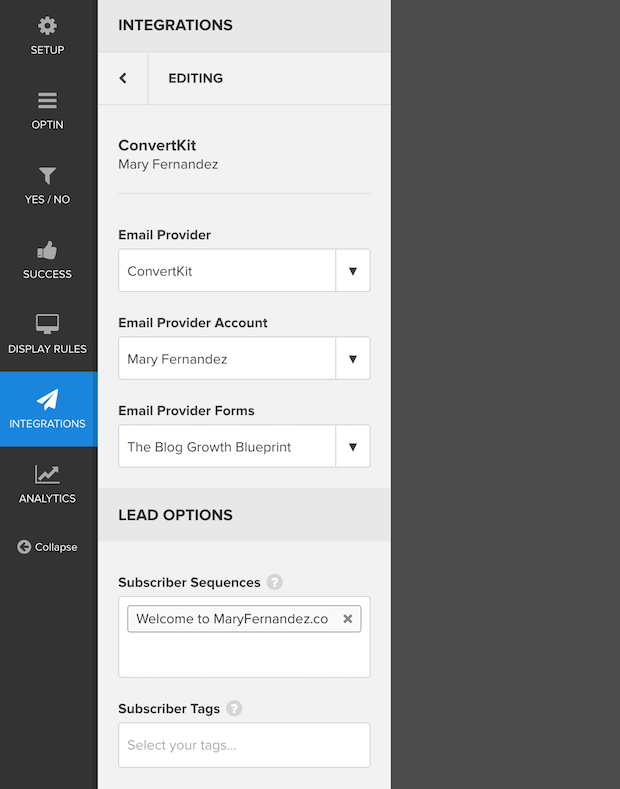The image displays a Setup or Integrations page with a dark-themed user interface, featuring a black background and white text for high contrast and readability. On the left-hand side, there is a vertical navigation menu with several icons and labels:

- **Setup** (gear icon)
- **Opt-in** (three horizontal bars icon)
- **Yes/No** (a glass or yes/no icon)
- **Success** (thumbs up icon)
- **Display Rules** (black and white monitor icon)
- **Integrations** (blue background, white text)
- **Analytics** (stock portfolio chart icon)
- **Collapse Menu** (left-pointing arrow icon)

The current page shown is the "Integrations" menu. The detailed section present under Integrations includes editing and managing integration settings for the email provider, Cover Kit, associated with the user Mary Fernandez. The available options in this section have various white boxes accompanying each item:

- **Email Provider Account**: Mary Fernandez
- **Email Provider Forms**: The Blog, The Growth Blueprint
- **Lead Options**
  - **Subscriber Sequences**: "Welcome to maryfernandez.co"
  - **Subscriber Tags**: Option to add tags to subscribers

To the right of this menu, there is a straight black bar devoid of any content or interactive elements, providing some empty space on the page.

This setup page is designed for users who are configuring their email and lead generation integrations, giving them an organized layout to manage different aspects of their email provider settings efficiently.